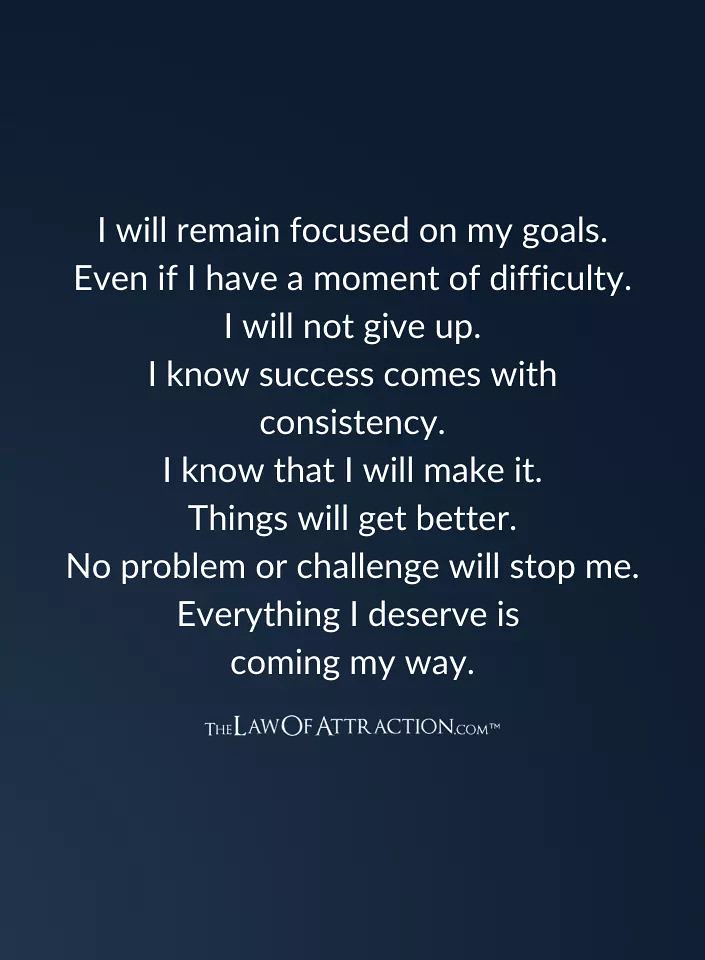The image features a rectangular design with a dark, solid blue background. At the center, a motivational quote is displayed in white print, arranged in multiple lines. The text reads: "I will remain focused on my goals. Even if I have a moment of difficulty, I will not give up. I know success comes with consistency. I know that I will make it. Things will get better. No problem or challenge will stop me. Everything I deserve is coming my way.” Below the motivational message, a URL in a smaller, slightly fancier font reads "TheLawOfAttraction.com," accompanied by a tiny "TM" in the top right corner of the 'M'. The entire composition utilizes only the colors dark blue and white, giving it a clean and focused appearance, making it suitable for sharing online or framing as an inspirational piece.